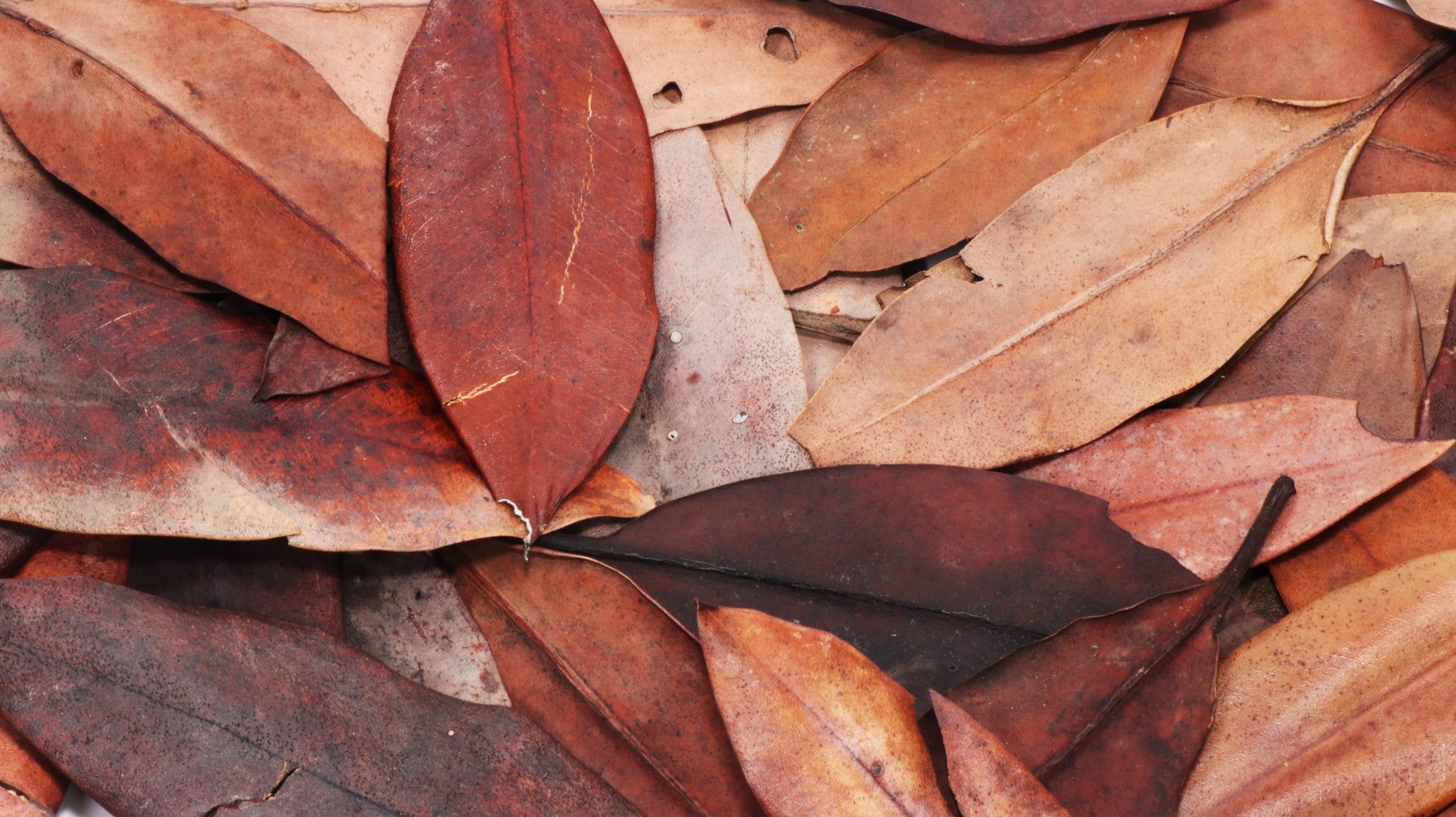The image depicts a close-up, outdoor scene of magnolia leaves that have fallen from the tree, now carpeting the ground so thoroughly that no grass or earth is visible. The leaves, their length around three to four inches, create a rich tapestry of autumn colors, ranging from dark reds, purples, oranges, and browns to bright reds, yellows with red speckles, and even some cream hues. All of them appear dry and crinkly, indicating they've been there for a while, with some showcasing holes, tears, and bites from small insects. The leaves are all scattered in various orientations—some right side up, others upside down. They feature classic, thinner shapes with distinct vertical veins running down the center and a diagonal vein pattern extending to the edges. The lighting is natural yet diffuse, suggesting an overcast day, and the overall composition of the image might give one the impression of an art student's careful arrangement.